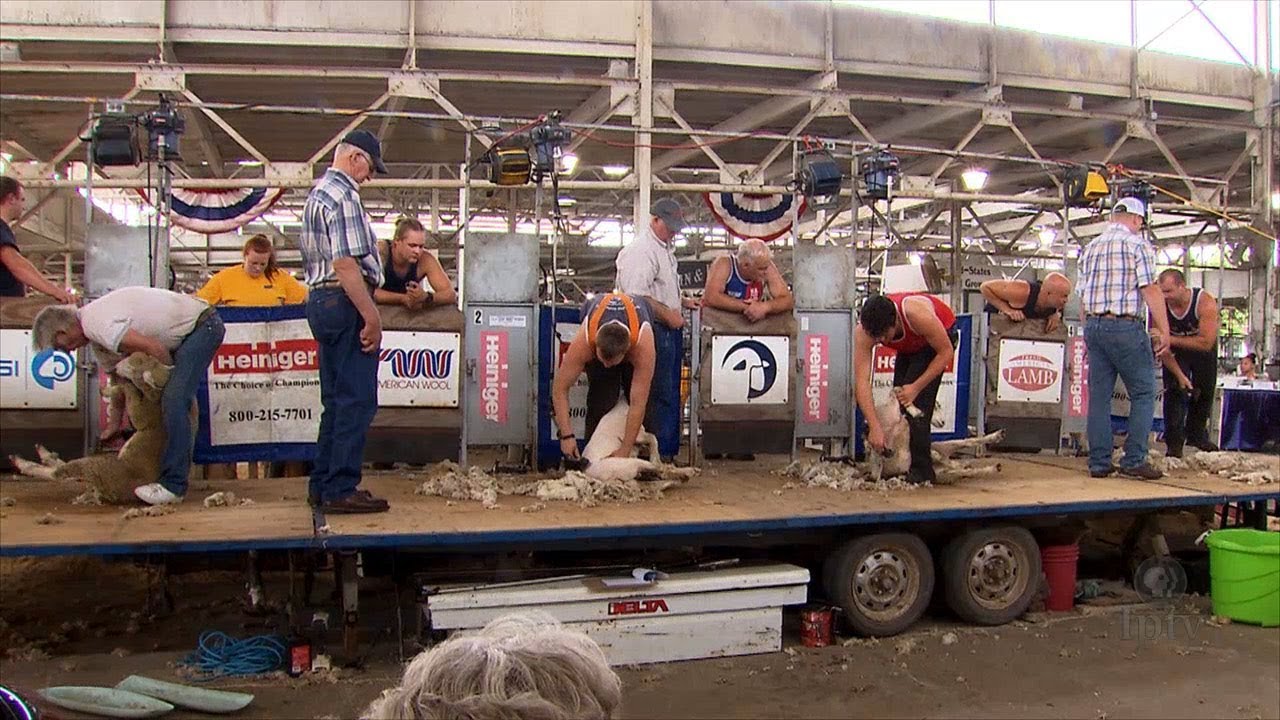In the image, a dynamic sheep shearing competition unfolds on a stage. Four male contestants, each diligently shearing their sheep, are the main focus. From left to right, the first contestant, an older man dressed in a white shirt and blue jeans, hauls a partially shorn sheep, leaning over a sign that reads "Heiniger, The Choice of Champions," with a phone number beneath. Behind him, a woman in a yellow shirt appears to be supporting him or holding the Heiniger sign.

Next, a man in blue jeans, a flannel shirt, and a blue cap, who likely serves as a judge, scrutinizes the efforts of the competitors. Adjacent to him stands another judge, an older man sporting a gray hat, a white shirt, and blue jeans, closely observing the third contestant. This contestant wears red suspenders over a blue shirt and blue jeans and is seen bending over a sheep almost entirely freed of its wool.

Amid the scene, a sign promoting "American Wool" is visible, guarded by a woman behind a gate, who might also be cheering on the participants. The fourth contestant, an older man in a gray hat, white shirt, and blue jeans, is captured mid-shear, his sheep nearly devoid of wool. To the right stands yet another sheep shearer, bald and clad in a sleeveless blue shirt, near a red sign with white writing that reads "Lamb." This individual's sheep is mostly obscured, visible only by one leg.

The spectators, friends, and family members are visible behind gated stalls, enthusiastically supporting their respective shearers. The ground is littered with a substantial amount of wool, indicative of the intensity of the competition. At the far right of the image, a green bucket and a white jack with red writing saying "Imella" rest beneath the stage, hinting at the event's logistical setup. Overall, the competitive atmosphere is palpable, with detailed sponsor signs such as "Heiniger" and "American Wool" adding to the authenticity of this robust sheep shearing contest.